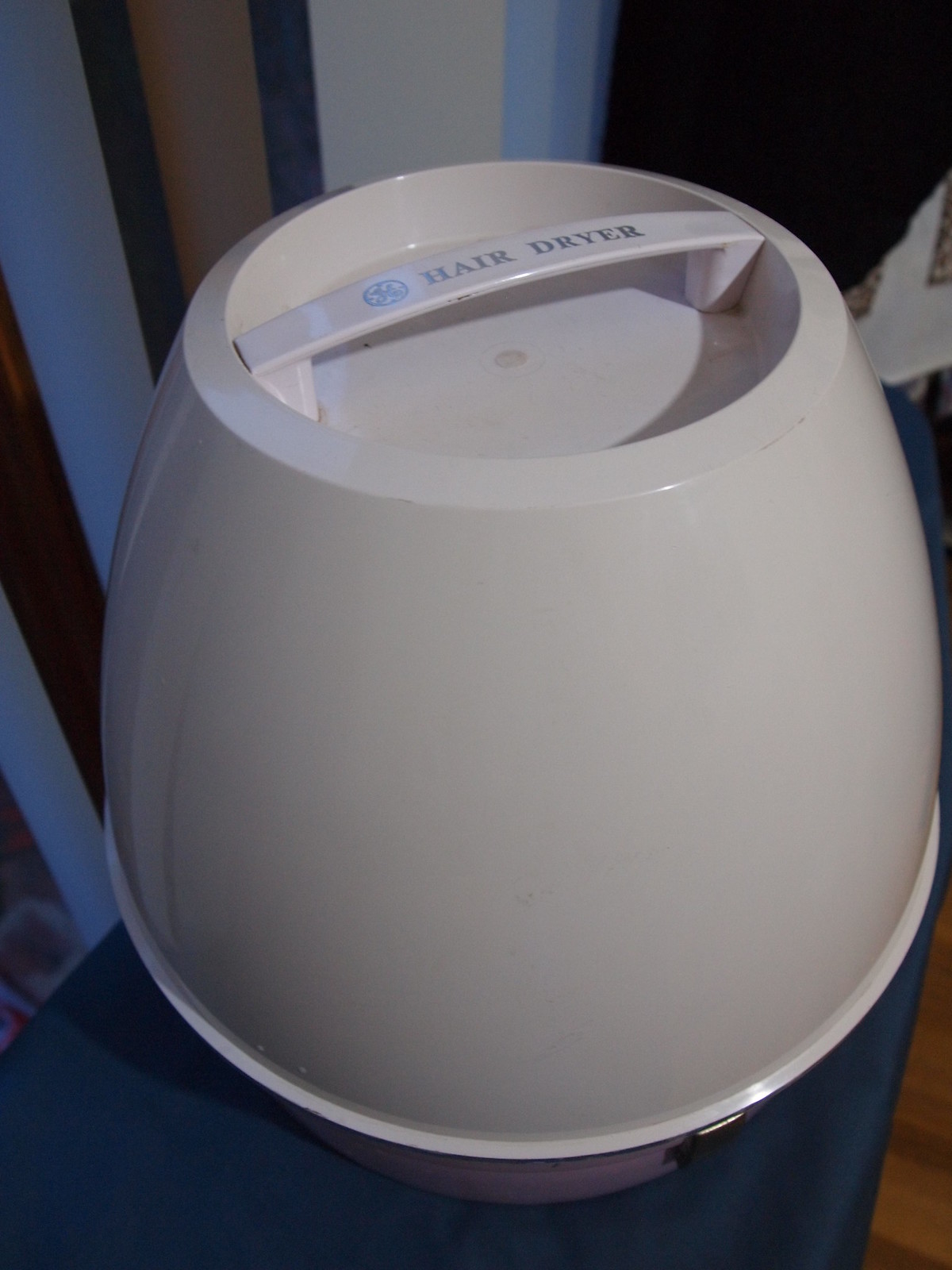The image features a rounded plastic case designed to store a hair dryer. The case prominently consists of a smooth white domed lid with a handle perched at the very top, which is inscribed with the words "hair dryer" in silver letters, accompanied by the GE logo. A small symbol is also visible next to the text. The bottom half of the case, which is slightly visible near the bottom of the image, is a pinkish hue and features a silver latch on the right side. The case is set upon a blue tablecloth, with a small portion of a wooden floor visible in the bottom right corner. The background includes a white wall with blue stripes running vertically and a black surface in the upper right corner.